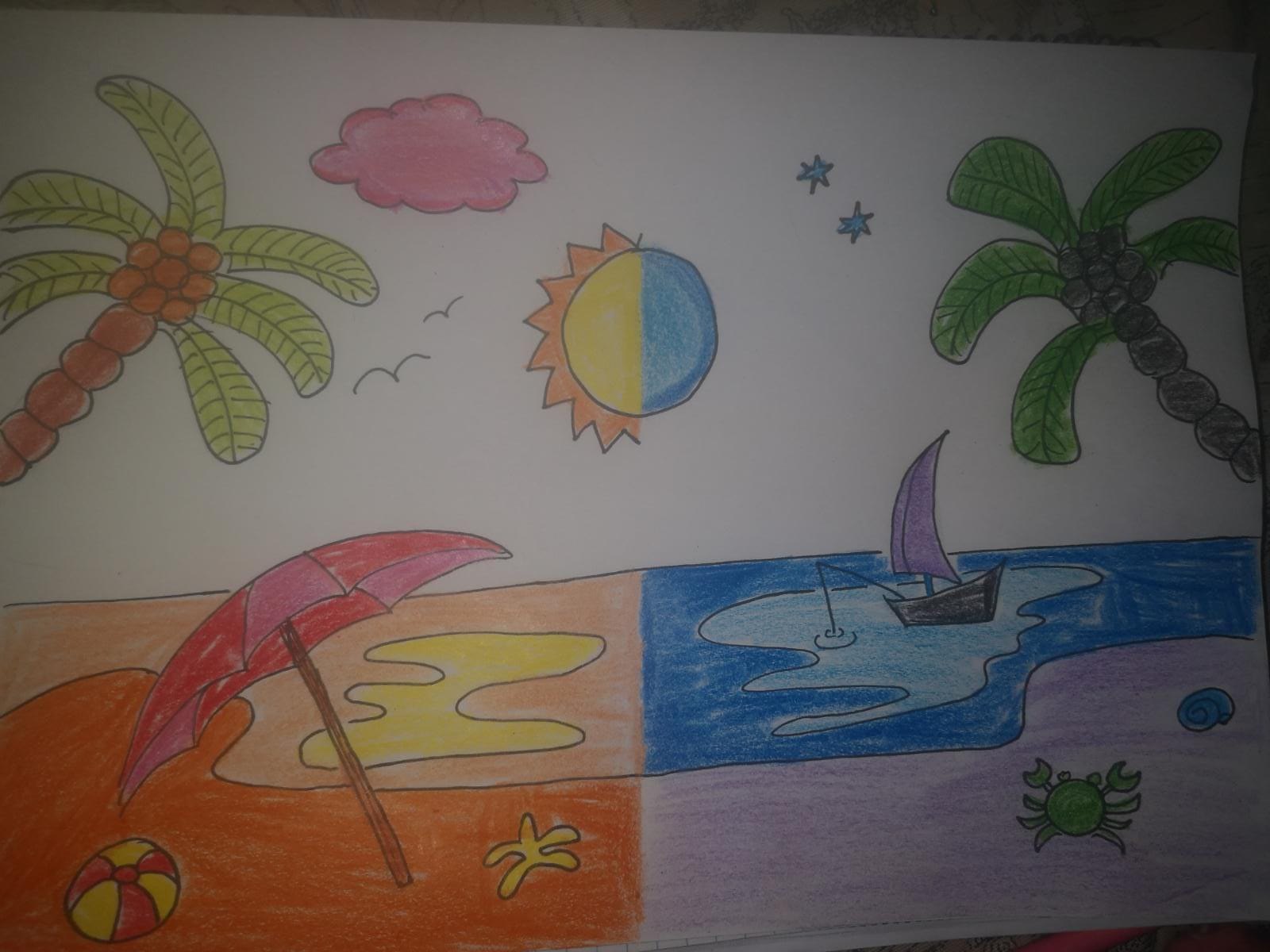The image is a detailed and vibrant drawing, possibly created by a middle school or high school student, or perhaps a slightly older child. It is divided into two contrasting scenes representing day and night on a beach. The drawing is on white paper and appears to be made with either crayons or colored pencils, featuring black pen outlines for definition.

On the left side, depicting day, the scene is bathed in warm colors. The sand is depicted in a rich orange, while the water shimmers in shades of orange and yellow. At the forefront, there is a red and pink beach umbrella leaning over the sandy beach, accompanied by a yellow and red beach ball and a yellow starfish. A tropical palm tree with a brown trunk and light green leaves also adorns this side. The sky includes a whimsical pink cloud and two outlined seagulls, alongside part of a sun that is half of a central circle, featuring yellow and orange rays expanding outward.

The right side of the drawing portrays night, using cooler tones. The water is depicted in different shades of blue, and the sand is colored purple. A palm tree with a grayish trunk and dark green leaves stretches into the scene. The night sky, left uncolored to show the white background, contains two blue stars and the other half of the central circle, representing the moon in soft blue hues. A small black sailboat with a purple sail floats on the water, and a fishing rod dangles overboard. On the beach, a green crab and a blue seashell are distinctly visible.

Overall, the image captures a split scene of a beach transitioning from the vivid warmth of day to the tranquil coolness of night, with intricate details and contrasting colors that highlight the difference between the two times of day.